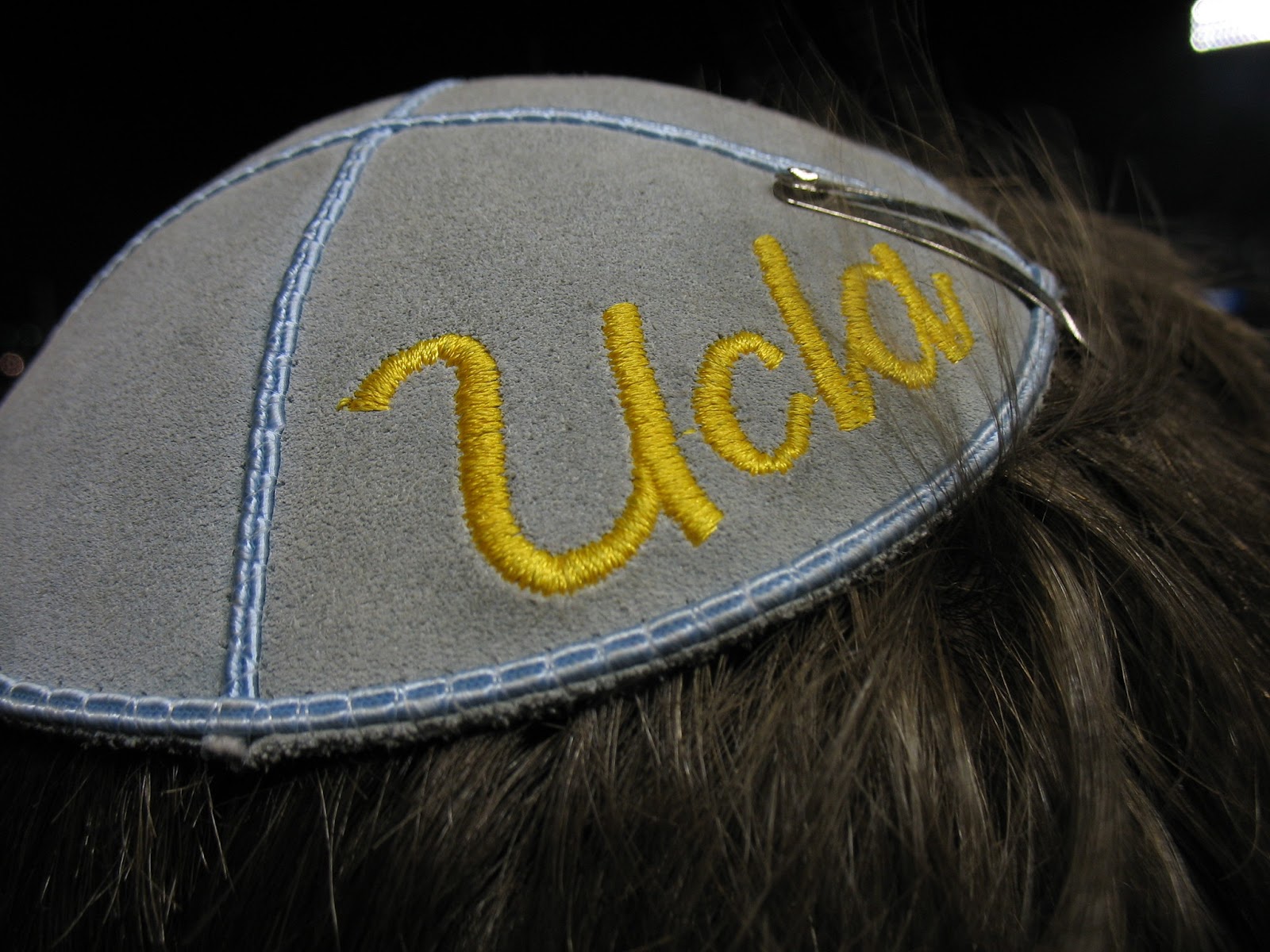This is a highly zoomed-in photograph of a man's head showcasing a yarmulke. The yarmulke, possibly made from gray suede or felt, is adorned with both vertical and horizontal baby-blue piping, as well as blue stitching along its perimeter. The standout feature is the yellow cursive embroidery of "UCLA" on one of its back quadrants, where the "U" is capitalized and "CLA" are in lowercase letters. The yarmulke is securely fastened to the man's short, dark brown hair with a simple silver metal hair clip. The image is very focused, offering no view of the man's face or surroundings, which are obscured by a dark black background.